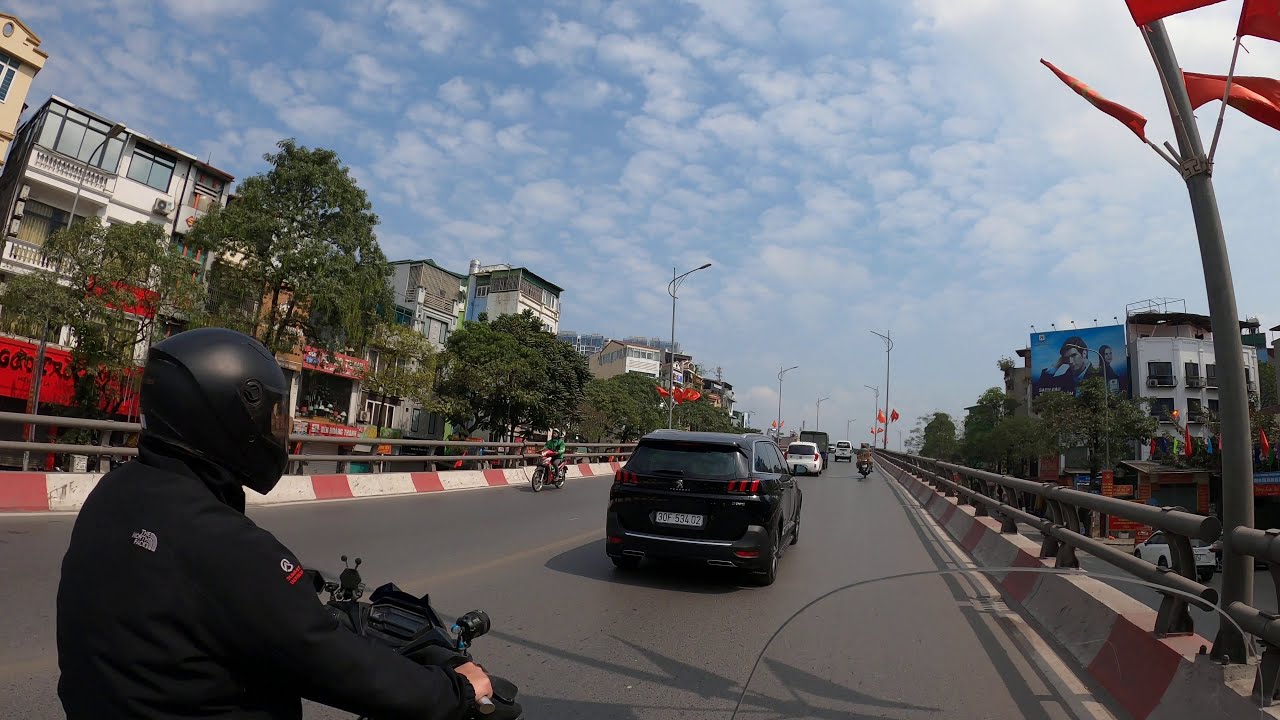A full-color, horizontally rectangular photograph captures a bustling street scene in a town on a mostly sunny day with a blue sky and light, fluffy cloud cover. Taken from the perspective of someone on a motorcycle, part of the windshield is visible in the bottom right corner. In the foreground, another motorcyclist wearing a black helmet and a long-sleeved black North Face jacket is seen riding a motorcycle. This motorcyclist is positioned to the left of the photographer. Ahead of them is a black SUV, and to the right, a white car. On the opposite side of the two-lane road, another motorcyclist on a red motorcycle wearing a green jacket is heading in the opposite direction. The road appears to be a bridge, flanked by gray metal railings with red and white painted concrete bases. The bridge stretches toward the background where orange flags suggest a construction zone. Street lamps line the road, and to the right, a large blue billboard featuring a person is displayed. The left side of the image reveals an assortment of three to four-story buildings, likely apartments, framed by trees, enriching the urban landscape.